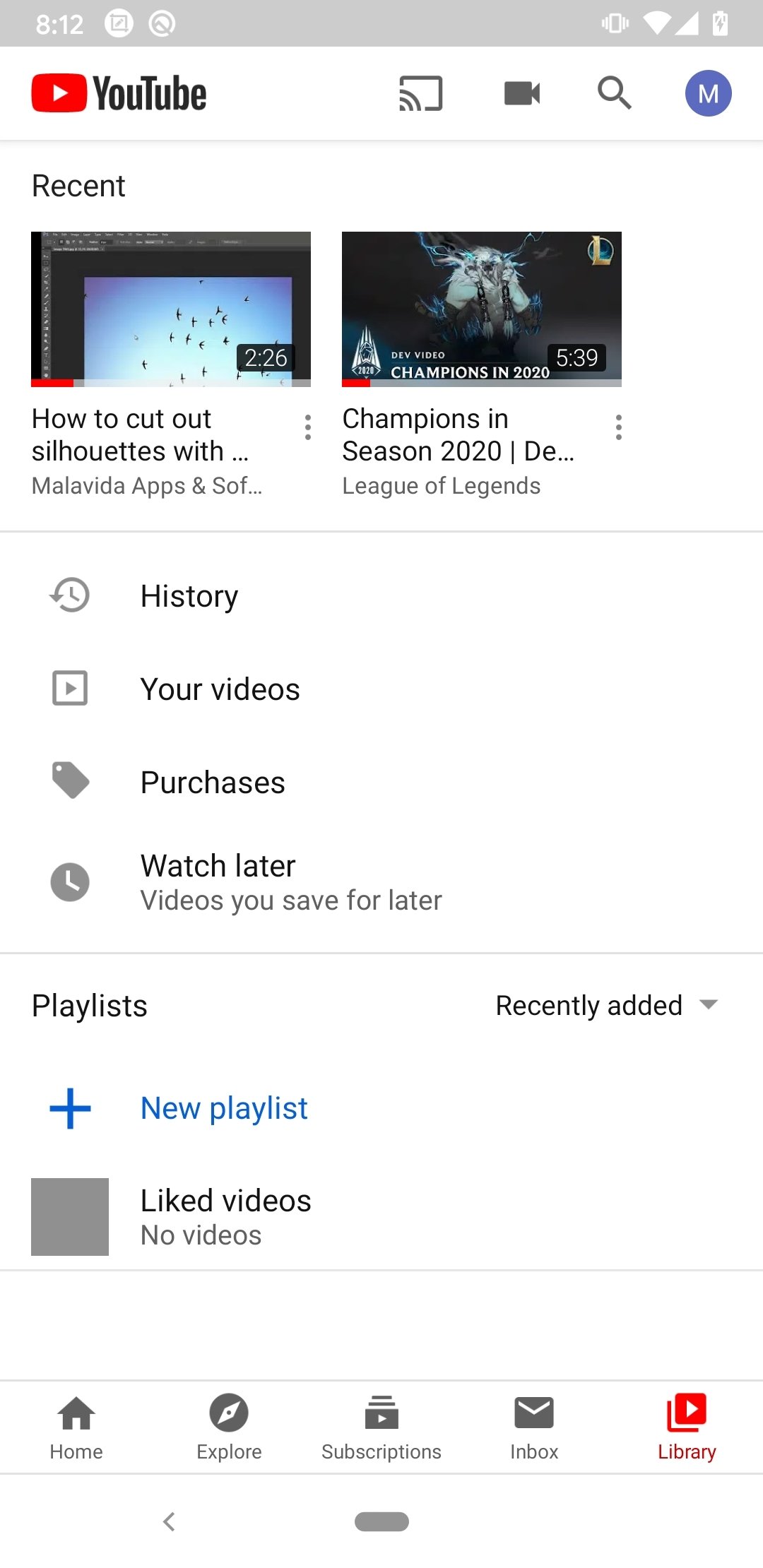This is a detailed smartphone screenshot of the YouTube app's user interface. On the top left corner, the screen displays the time as "8:12" within a gray status bar. In the upper right corner, common smartphone icons for internet connectivity and battery power are visible.

At the top of the YouTube app interface, you see the YouTube label along with its recognizable red rectangle logo featuring a white play button inside. Below this, a section labeled "Recent" shows two video thumbnails. The first thumbnail on the left depicts a sky filled with birds accompanied by the partially visible title "How to cut out silhouettes with…". The second thumbnail on the right displays a creature in chains, with the accompanying title reading "Champions in Season 2020 | League of Legends".

Further down, the screen features a horizontal menu bar with various options. There's a small clock icon next to the word "History", a square icon with a triangle labeled "Your Videos", a price tag icon with "Purchases", and another clock icon indicating "Watch Later" for saved videos. Below this section, a dividing line separates these functions from the "Playlists" section.

In the "Playlists" section, there’s a blue plus sign next to the text "New Playlist" for creating new playlists. Below this, a gray square indicates "Liked videos" with a note stating "No videos."

At the bottom of the screen, a navigation bar contains icons for "Home," "Explore," "Subscriptions," "Inbox," and "Library." The "Library" icon is highlighted in red, while the others remain in gray, suggesting the current active section.